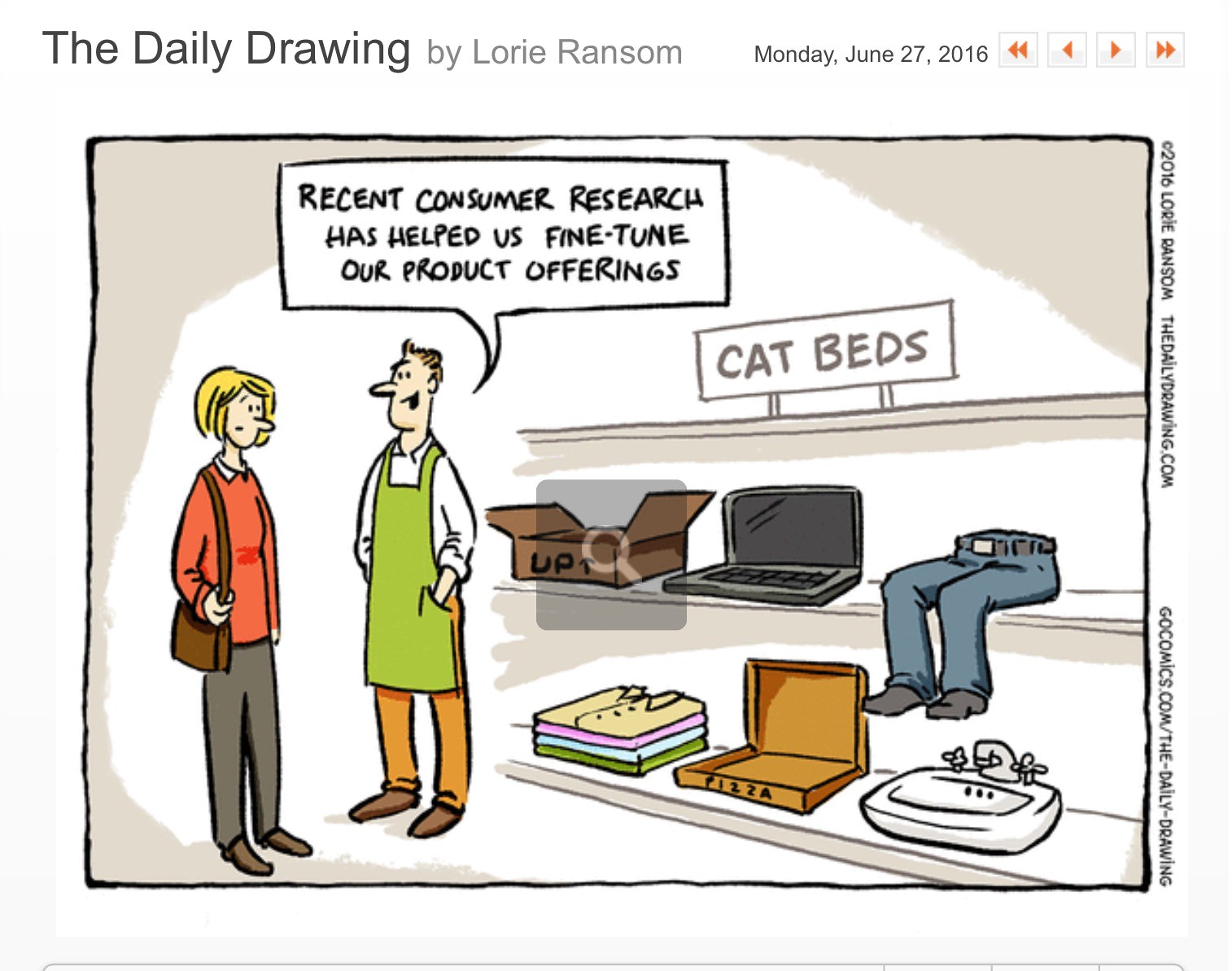In a single comic strip panel titled "The Daily Drawing by Lori Ransom, Monday, June 27th, 2016," a woman and a man are depicted having a conversation in what appears to be a store. The woman, with short blonde hair, is wearing a red long-sleeve shirt with a white collar, grey pants, brown shoes, and a brown purse over her shoulder, indicating she might be shopping. The man, who looks like a shopkeeper, has short blonde hair and is dressed in a white collared shirt, tan pants, brown shoes, and a lime green apron. He is speaking to the woman, with a speech bubble above his head reading, "Recent consumer research has helped us fine-tune our product offerings." 

Behind the man are shelves labeled "cat beds," which humorously contain items that cats typically enjoy sitting on: a cardboard box, a laptop, a pair of jeans with feet but no torso, a pile of folded shirts, an opened pizza box, and a white ceramic sink. The scene cleverly mocks the eccentric preferences of cats in a retail context.